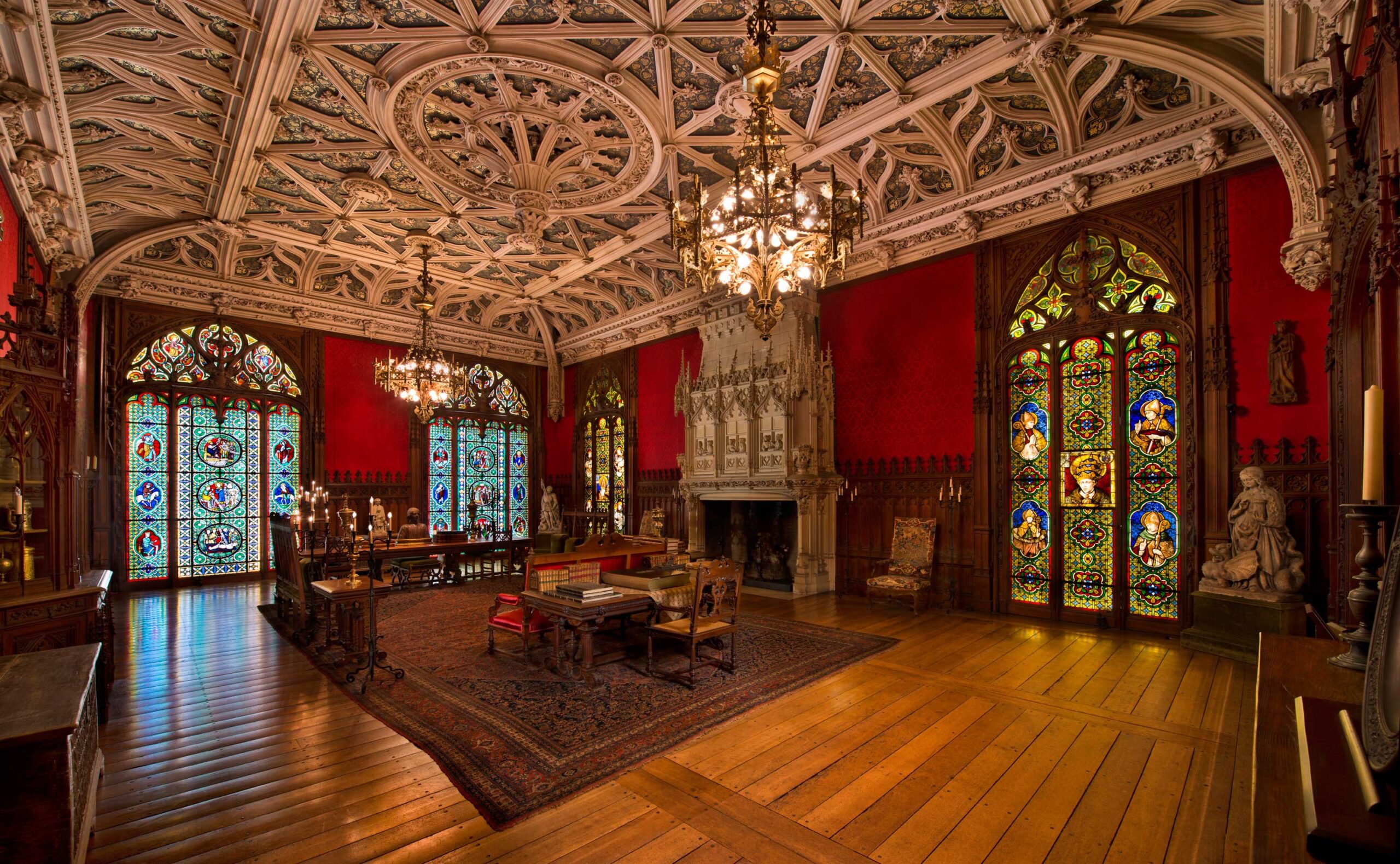This image depicts an opulent and intricate room, evoking a historical or cathedral-like ambiance. The decor is characterized by a richly embossed ceiling featuring white ornamental florets and branching arches, from which hang grand chandeliers. The room's walls are a deep burgundy hue, providing a striking contrast to the extensive use of various wooden elements, including large plank floors and wood filigree throughout the ceiling.

The room boasts several stunning stained glass windows, featuring intricate designs and depicting people, biblical scenes, and equestrian figures. Two windows are predominantly blue, and two are green, enhancing the room's vibrant palette that includes shades of blue, green, burgundy, and silver.

A prominently aged and unlit white fireplace is situated in the middle back of the room, accompanied by a chair and decorated with surrounding objects. To the right, a statue stands among various food items, while a piece of furniture with a candlestick is positioned nearby.

The room is furnished with multiple items: a central ornate rug with a desk and chair set up for study, additional coffee tables scattered around, a dining table surrounded by chairs, and statues and busts placed throughout. A table with lit candelabras and books signifies a space designed for both grandeur and functionality. The overall effect is one of elaborate detail and historical elegance.